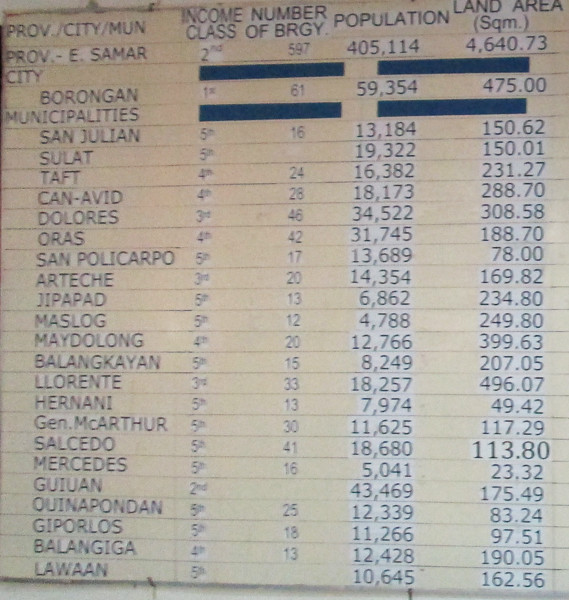The image showcases a detailed chart or table in the form of a poster or card with a tan, white, and bluish color scheme. The primary object of the image is the page itself, which lists demographic statistics of various cities and municipalities in the province of Eastern Samar. The left column is labeled 'Province/City/Municipality' and it features names such as Borongan, San Julian, Salat, Taft, Can Avid, Dolores, Oris, San Policarpo, Arteche, Jipapad, Maslog, Maydolong, Balangiga, Llorente, Hernani, General MacArthur, Salcedo, Mercedes, Guiuan, Quinapondan, Giporlos, and Lawaan among others. The additional columns provide data under headings like 'Income Class', 'Number of BRGY', 'Population', and 'Land Area'. The style of the document suggests it is a printout detailing demographic and administrative statistics for the various locations within Eastern Samar.